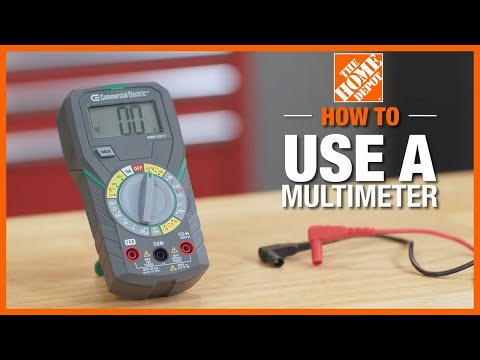The image is a detailed Home Depot instructional poster set against a black background, featuring prominent text and a multimeter on a wooden table. The top and bottom of the poster are bordered with black horizontal strips, framing an inner orange rectangle. Within this rectangle, on the right side, the Home Depot logo in white letters is prominently displayed within a square. Below the logo, "How To" is written in bold orange letters, followed by "Use a Multimeter" in white letters.

On the left side of the table, there is a gray multimeter with a digital readout at the top displaying "00." Below the digital screen, a circular dial is present, marked with various colors such as gray, yellow, white, and red, each corresponding to different settings. This dial allows the user to select different measurement modes, though specific numbers and settings are not clearly visible due to blurriness. Beneath the dial, there are three plug-in ports: two red ports on the outer sides and a black port in the center, with lines and numbers indicating their functions.

To the right of the multimeter, two electrical cords, one red and one black, are visible, suggesting their use in conjunction with the multimeter. The background is slightly blurred but shows additional hints of red, gray, and black colors. This entire scene is captured indoors on a light brown wooden table, providing a subtle yet effective contrast to the device and the instructional text.

The carefully structured layout and color coordination make the poster visually appealing and clear, aimed at guiding users on the proper use of a multimeter.